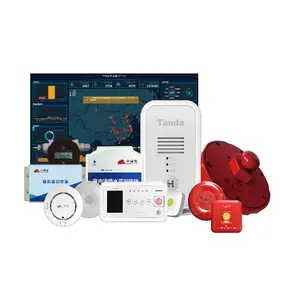The image presents an advertisement for a weather system alarm branded as "Tanda". Centered against a plain white background, the ad showcases a collection of electronic devices. Prominently displayed is a red siren with a red button, alongside a wall-mounted white device that likely monitors air or environmental conditions, accompanied by a thermostat-like device. The group also includes a white gadget with a small screen and buttons, resembling an air conditioning control unit. Arranged around these main items are several smaller electronic components and round objects, both white and red, that hint at various functionalities. A background screenshot of a website or application features a map dotted with red points, adding context to the device's purpose. The image lacks any boundary or text, focusing solely on the array of devices that appear to be designed for monitoring and alerting within a comprehensive system.